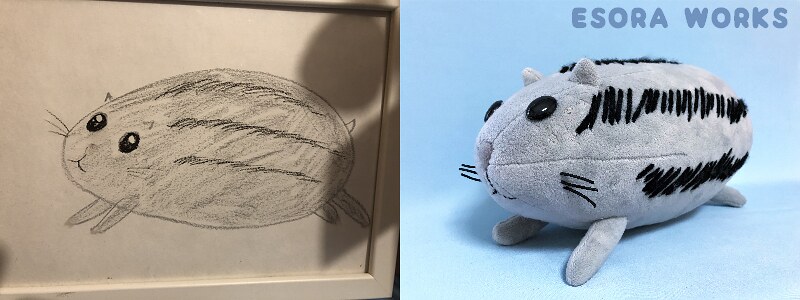On the left side of the image is a highly detailed black and white sketch, remarkably realistic, capturing the intricate details of the subject depicted on the right side. The right side features a photograph of a small, adorable stuffed animal, resembling a realistic, furry collectible. This plush toy has lifelike black whiskers and a textured gray coat that gives it an incredibly authentic appearance. The attention to detail on the toy's facial features, particularly the whiskers and strands of hair, adds to the overall cuteness and realism of the piece. In the top right-hand corner of the right side, the logo "Sora Works" is displayed on a blue background, lending an artistic and professional touch to the image. The sketch on the left is an impressive replication of the photograph, so much so that the pencil rendering almost appears more real than the live photo.